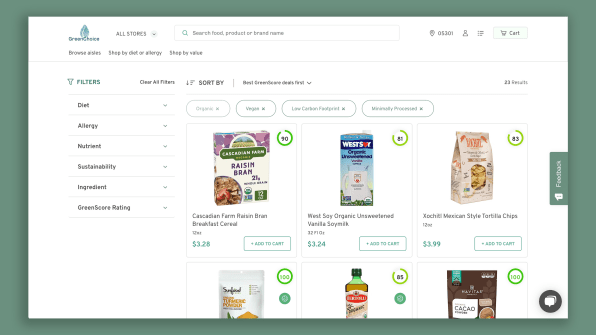This image is a screenshot from a shopping website, characterized by a distinctive layout and various navigational elements. The top and bottom borders feature a dark green band approximately a quarter inch in thickness, while the left and right sides have a matching dark green border about an inch wide. 

In the center, the background is white, providing a clean look for the main content. At the top left corner, there's a somewhat blurry green leaf icon accompanied by the text "Green Choice" in black. To its right, a dropdown tab labeled "All Stores" can be found. 

The central part of the header contains a lengthy search bar, about four inches wide, with a search icon inside and placeholder text that reads, "Search food, common product, or brand name." On the right side, a light blue tab displaying "Cart" in black, alongside a cart icon, is prominently visible. Additionally, an account section exists with an icon, the numbers "05301," and three horizontal lines accompanied by a dot on the left side.

On the left side of the screen, the options "Browse Aisles," "Shop by Diet or Allergy," and "Shop by Value" are listed in black text, though the text appears blurry. Below this section is a black bar, and beneath that, there's a blue filter section labeled "Filters," followed by six dropdown tabs. The rightmost tab is labeled "Clear All Filters," with another dropdown tab to its right.

Further right, the text "Sort by" appears, with yet another dropdown tab adjacent to it. Below the "Sort by" section is another label, "23 Default." 

The main part of the page showcases various products for purchase. At the top, there are four rectangular white buttons with black text, indicating clickable options. Below these buttons are three product listings, each displaying a picture of the product, the product name beneath it, the price in the bottom left corner, and an "Add to Cart" button in the bottom right corner. Additionally, there is a half-green circle with numbers indicating some form of metric or rating.

Finally, below these three products, three more product images are partially visible, completing the browsing section of the screenshot.